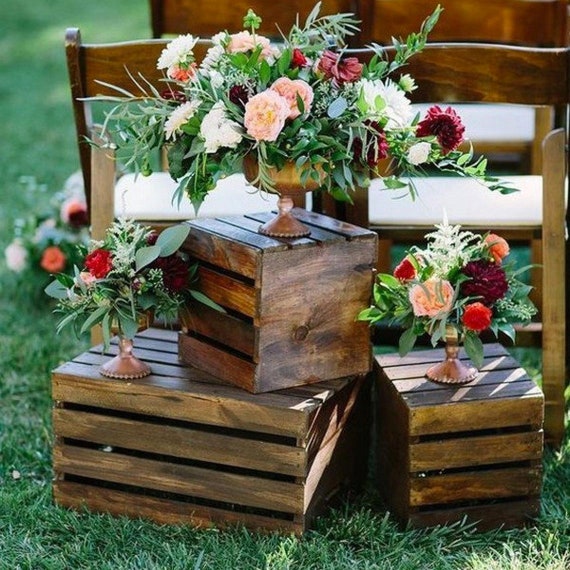In this outdoor scene, the grass-covered ground features an arrangement of three dark-stained wooden crates, reminiscent of old-style milk boxes. The largest crate, rectangular and broad, rests directly on the ground, with a smaller square crate placed on top of it, and another smaller square crate positioned separately. Each crate is adorned with a decorative bronze-colored vase, each holding a bouquet of flowers in varying shades of pink, white, and maroon, accentuated by lush greenery. Behind these crates stand two wooden chairs equipped with white seat cushions, and nestled between the chairs and the crates are additional bouquets of flowers lying on the grass. The backdrop is completed with glimpses of light brown wooden posts and hints of more chairs in the distance, contributing to the serene and rustic ambiance of the image.